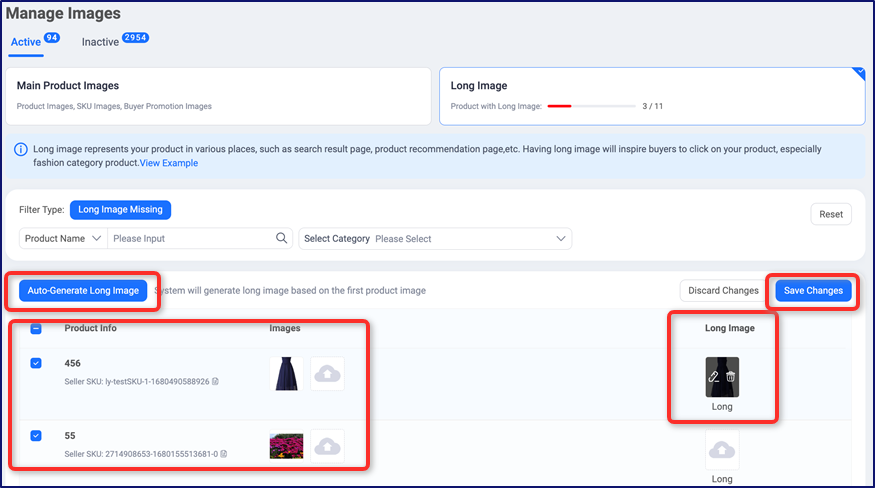The screenshot depicts a web interface designed for managing product images on an e-commerce platform. The top section of the page displays a navigation menu with options such as 'Manage Images,' which shows the counts for 'Active' (94) and 'Inactive' (2954) images. There are also specific image categories including 'Main Product Images,' 'Long Image,' and 'Long Image Missing,' with an option to 'Auto-Generate Long Image.'

Prominently featured on the lower left is a section titled 'Product Info and Images,' which displays 456 Seller SKUs and 55 Seller SKUs, indicating a detailed inventory management system. The platform appears to facilitate sellers in uploading and managing images for their products, ensuring buyers can view visual representations of the items listed for sale. This functionality is integral to optimizing the online shopping experience, enabling sellers to create SKUs and present comprehensive product visuals to potential buyers on their e-commerce pages.